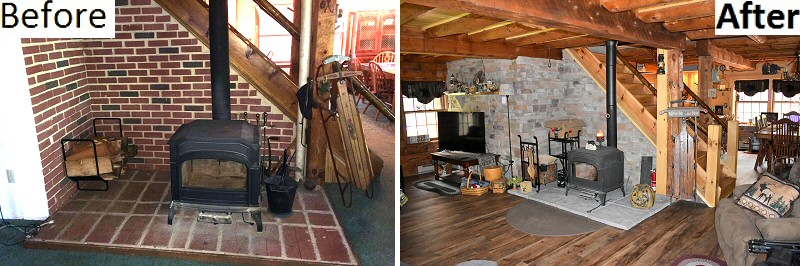The image showcases a before-and-after comparison of a remodeled wall section around a wood-burning stove, captured in two side-by-side rectangular photos. The left-side image, labeled "Before," features a black wood stove set against a backdrop of old brickwork comprising brown, black, and white bricks. The wood stove rests on a platform of large red bricks, surrounded by dark green carpeting. Visible to the left of the stove is the edge of a wooden staircase and a white wall with an electrical outlet, bookshelves, and a partial view of a table. Additional details include a wood rack with logs and a black flue extending from the stove upward, presumably through the ceiling.

In the "After" image on the right, the room has undergone significant changes. The original brick backdrop has been replaced with a stone veneer in tones of white, black, and red. The large red bricks beneath the stove are now substituted with large white blocks, and the flooring has transitioned from green carpet to dark brown wood laminate. The staircase is seen from a different angle, revealing the steps more clearly, and appears to be made of a lighter, brighter wood. The room also now includes a flat-screen TV, additional rugs, and seating, indicating it serves as a living room. The ceiling consists of dark brown wood beams and wooden panels, complementing the rustic theme of the remodeled space.